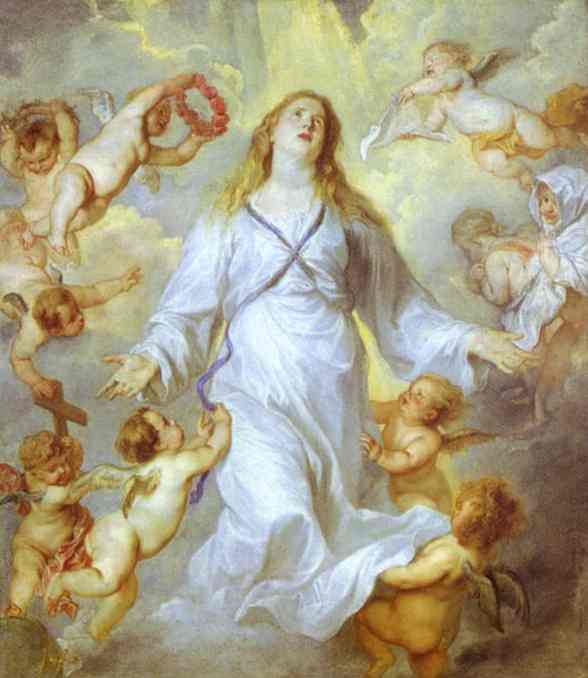The image is a vertical rectangular religious painting featuring a central figure of a woman in a long, flowing white gown with gold straps across the top. She has long, light brown to blonde hair and red lips. Her arms are gracefully spread out in front of her, palms up, as she faces us while looking upwards. Surrounding her are numerous winged cherubs, all of whom are naked apart from their wings in varied colors, with some depicted with halos. One cherub, located on her left, seems poised to place a red decorative ornament or a beaded necklace on her head. Another cherub near this one is presenting a wooden cross. A cherub at the bottom right of her gown clutches the fabric while looking up at her. The backdrop of the painting blends shades of gray, brown, and white, with a bright, shining light emanating from the top amidst a cluster of clouds, creating a divine ambiance.